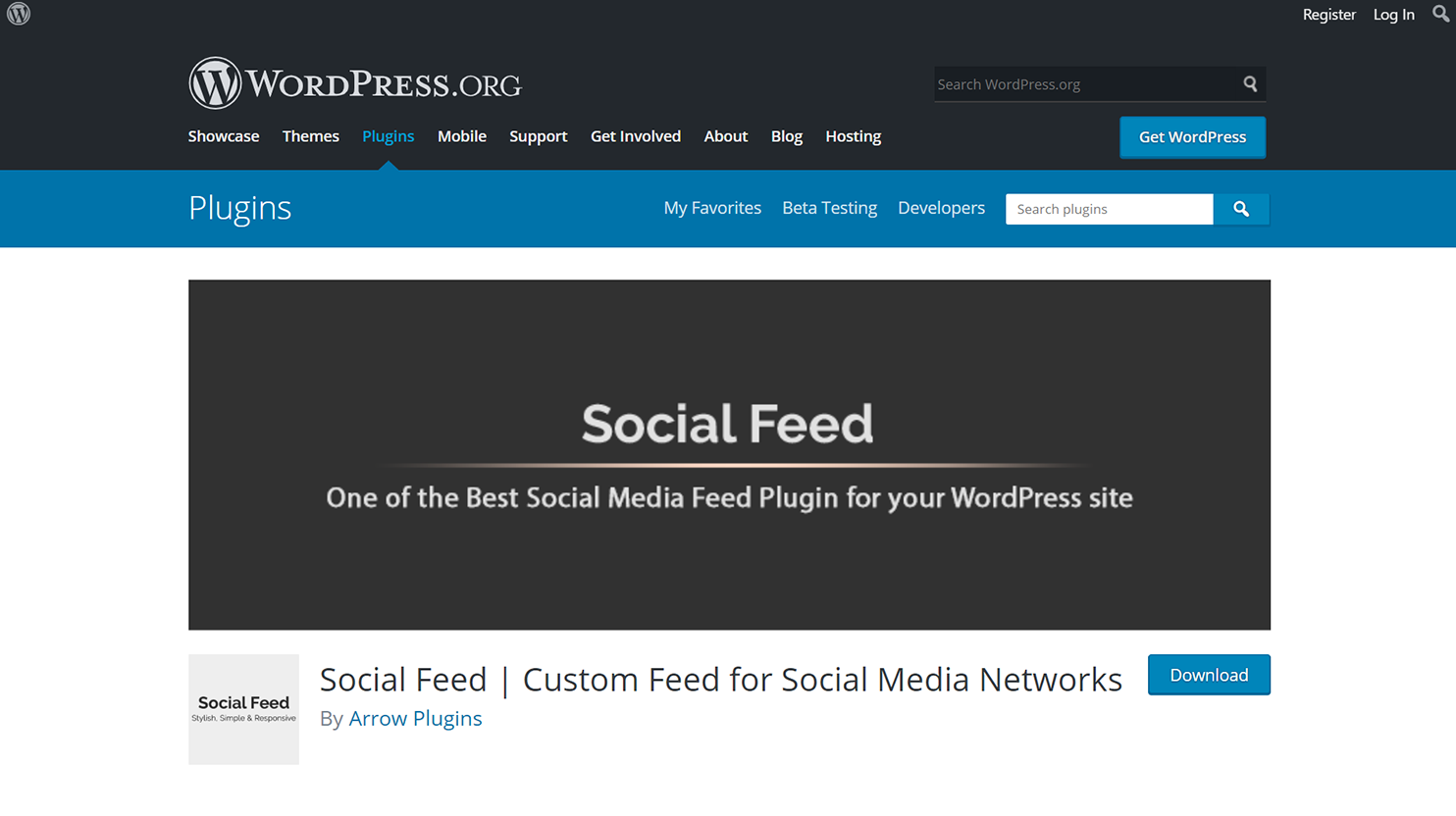Screenshot from the WordPress.org Website:

At the top of the screenshot, there is a rectangular black banner. In the far upper left corner, the black and white "W" WordPress logo is displayed. On the upper right corner of the banner, there are links in white text: "Register," "Login," and an icon of a magnifying glass representing the search function. 

Towards the left side of the banner, a larger version of the black and white WordPress logo is visible. To the right of this logo, the text "WordPress.org" is prominently displayed in bold white letters. Below this, a navigation menu is present with links in white text: "Showcase," "Themes," and a currently selected "Plugins" link, which is highlighted in blue. The continuation of the navigation line includes: "Mobile," "Support," "Get Involved," "About," "Blog," and "Hosting."

Positioned slightly upward at around a two o'clock direction, there's a black search bar with a white magnifying glass icon beside it. Below the search bar, there's a blue button with white text that reads "Get WordPress."

Beneath this section, a sky blue banner appears. On the left side of the banner, in white text, the word "Plugins" is displayed. To the right, additional white text reads: "My Favorites," "Beta Testing," "Developers," along with another search bar and a magnifying glass icon.

The central area of the screenshot features a large black rectangle. Centered within this rectangle, bold white text states "Social Feed." Directly underneath, a pinkish line is followed by smaller white text that reads: "One of the best social media feed plugins for your WordPress site."

At the bottom of the image, against a white background, there's a gray square on the bottom left containing the text "Social Feed." To the right of this, it reads: "Social Feed - Custom feed for social media networks." Further to the right, there’s a blue rectangular download button with white text that says "Download." Directly below "Social Feed" on the left side, it’s indicated in blue text that the plugin is by "Arrow Plugins."